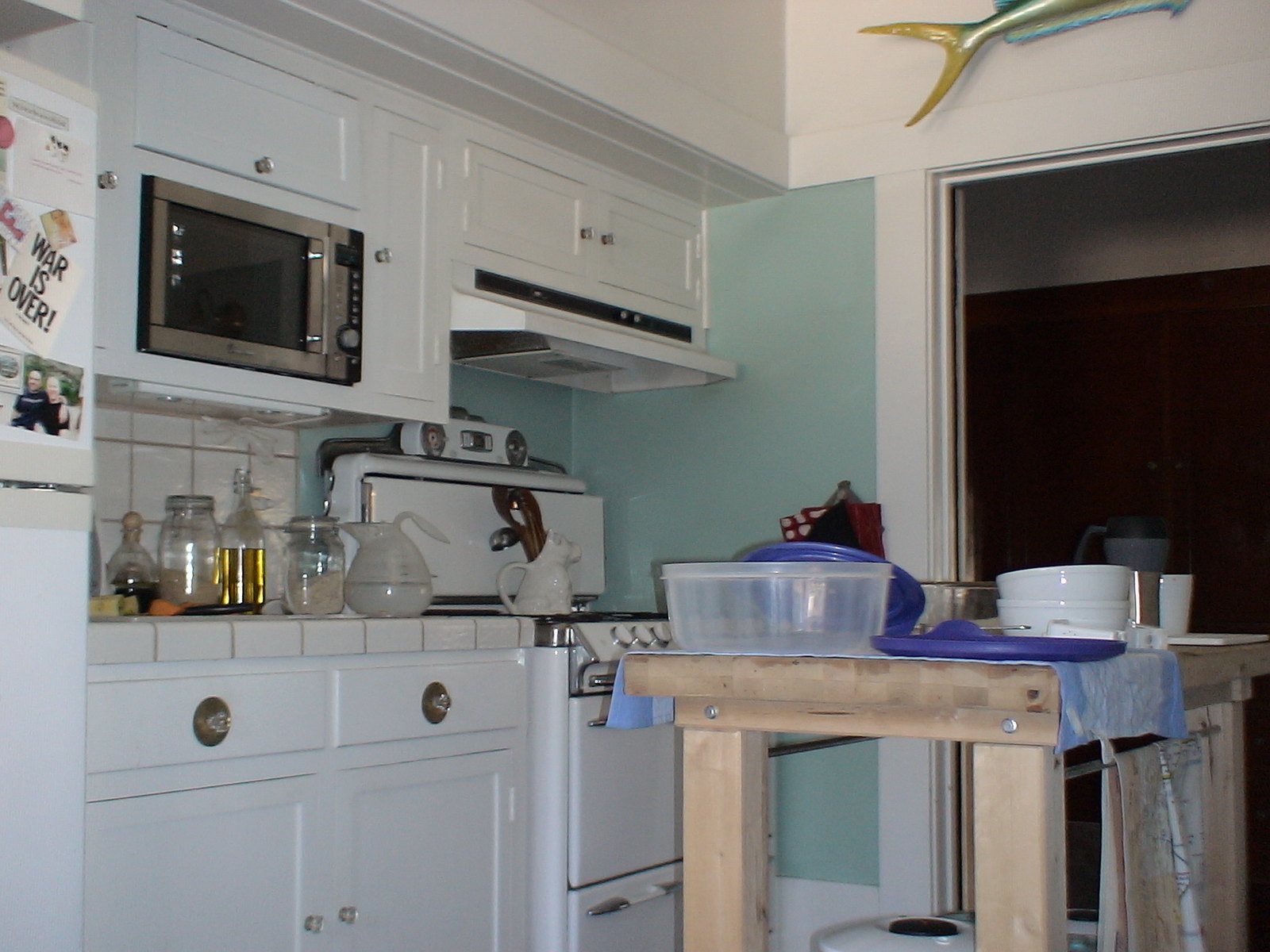This photograph captures a bright and inviting kitchen area, featuring a centerpiece kitchen island made of blonde-colored wood. The island is supported by sturdy, two-by-four legs, bolted together to form a solid countertop. Draped across the island is a blue and white patterned towel, on which a set of Tupperware containers with purple lids, white ceramic bowls, and a gray thermos are left out to dry.

The kitchen walls are primarily painted white, framed by a white border that leads into an adjoining room with brown doors. Hanging partially within the frame is the yellow tail of a fish mounted on the wall, adding a touch of whimsy to the space. The wall behind the stove and oven boasts an aquamarine color, complementing the retro-styled white appliances with their silver metal accents. A modern silver microwave is seamlessly integrated into the white cabinetry, which features clear glass knobs, adding a touch of elegance.

Below the microwave, white cabinets and drawers continue the theme, topped with a white tile countertop. This countertop is adorned with various pitchers filled with liquids and canisters filled with ingredients like flour, neatly arranged to indicate a well-used and organized kitchen space.